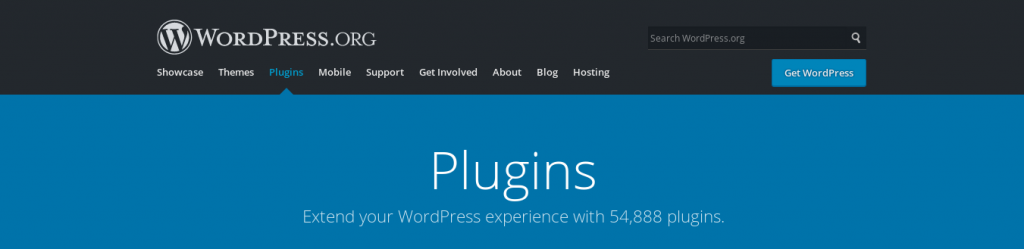A partial screenshot of the WordPress.org website showcasing its interface. The top banner is black, featuring tabs for "Showcase," "Themes," "Plugins," "Mobile," "Support," "Get Involved," "About," "Blog," and "Hosting." Below the banner is a blue section with a prominent blue button labeled "Get WordPress." At the top, there is a search bar with the placeholder text "Search WordPress.org" and a magnifying glass icon.

The "Plugins" tab is selected, revealing text in white that states, "Extend your WordPress experience with 54,888 plugins." This highlights the extensive range of plugins available to enhance the functionality of WordPress websites. WordPress.org is renowned as a platform where users can publish blogs, articles, and multimedia content. It caters to individual bloggers, small businesses, and larger corporations, serving as a versatile tool for a wide range of online publishing needs. The availability of 54,888 plugins underscores its popularity and the vast customization options it offers to its users.